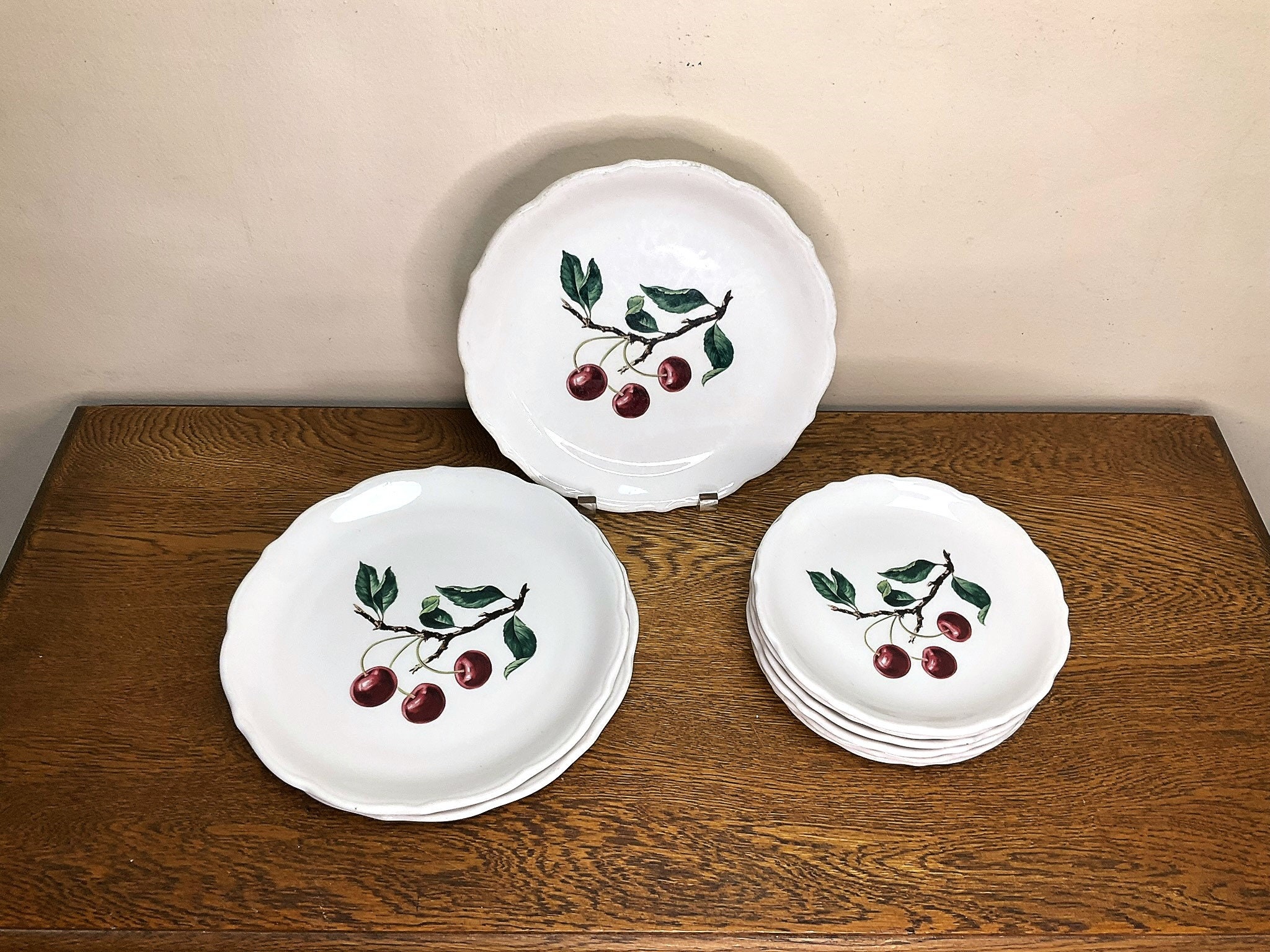This photograph depicts a beautifully arranged setting featuring elegant porcelain plates on a dark wooden table, set against a light gray wall. Centrally positioned, one plate with a delicate scalloped edge is held upright in a stand. Each plate showcases a charming design of a cherry tree branch adorned with leaves and three vibrant, bright red cherries. To the left of the upright plate, there is a stack of two larger, dinner-sized plates, while on the right, there is a stack of five smaller plates, possibly for bread. Both stacks of plates share the same intricate cherry branch motif, creating a cohesive and visually pleasing display.